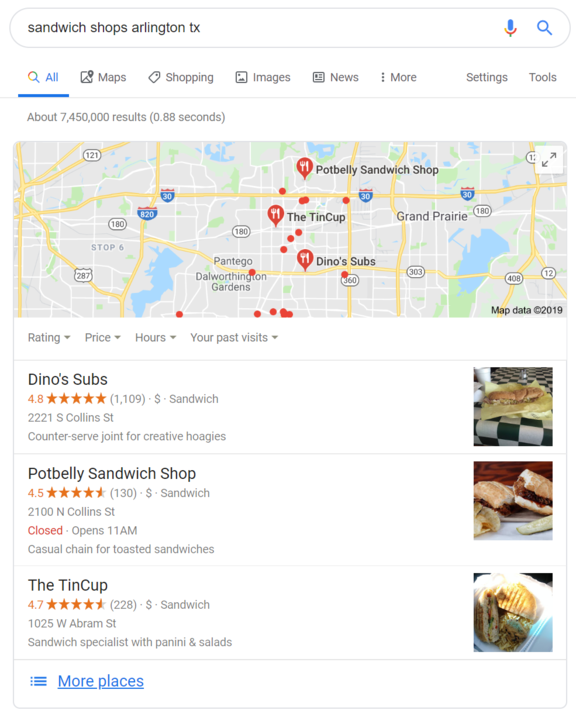This image displays a search results page for "Sandwich Shops, Arlington, Texas." At the top, the search bar highlights the query, and the "All" tab is selected. Below the search bar, a detailed map showcases various streets, some highlighted in yellow, with a few red pins marked with a white fork and knife symbol, pinpointing specific restaurants. These restaurants include Potbelly Sandwich Shop, the Tin Cup, and Dino's Subs. The bottom right corner of the map notes, "Map Data ©2019."

Underneath the map section, the categories "Rating," "Price," "Hours," and "Your Past Visits" are listed. Three search results are presented:

1. **Dino's Subs**: Rated 4.8 stars, this listing includes the address and describes it as a counter-serve joint for creative sandwiches. On the far right, a photo displays a sandwich atop a wrapper on a black and white checkered tablecloth.

2. **Potbelly Sandwich Shop**: Receiving 4.5 stars, the listing shows the address and notes it is currently closed, reopening at 11 a.m. It is described as a casual chain for toasted sandwiches. The accompanying photo features a sandwich cut in half.

3. **The Tin Cup**: With a rating of 4.7 stars, the address is listed along with a description of the establishment as a sandwich specialist offering paninis and salads. The adjacent photo is a close-up of a cut sandwich.